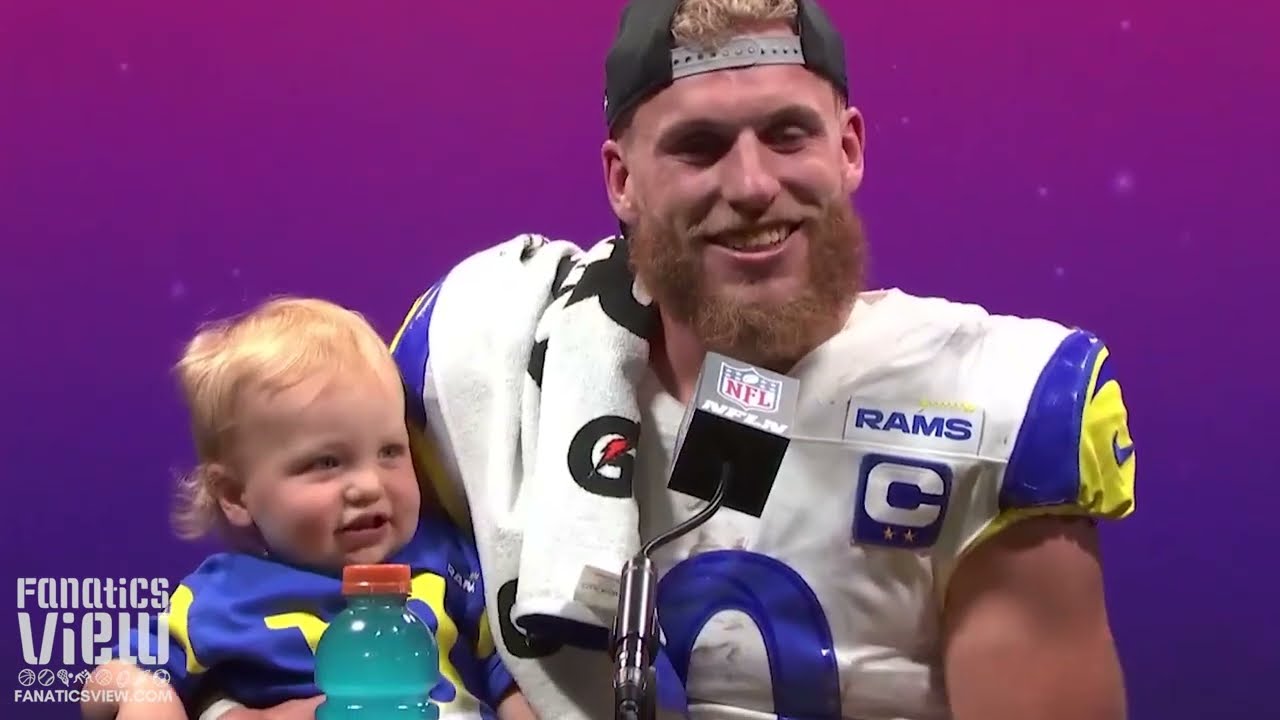In a wide, rectangular image, a professional football player, dressed in a blue and white Rams uniform, stands with a smile, holding his toddler son. The man, who has white skin and a red beard, sports a backwards black baseball cap and is positioned to the right side of the frame. An NFL microphone is seen in front of him. The child, with blonde hair, wears a blue and yellow shirt and is held in the player's right arm, looking off to the right. Both stand against a vibrant background that transitions from magenta at the top to purple at the bottom, scattered with faint white dots resembling stars. The football player also has a Gatorade towel draped over his shoulder and a blue Gatorade bottle with an orange top is visible on the podium in front of him. In the bottom left corner of the image, the text "FANATICS VIEW" appears prominently in white letters, along with several sports symbols and the website "fanaticsview.com".